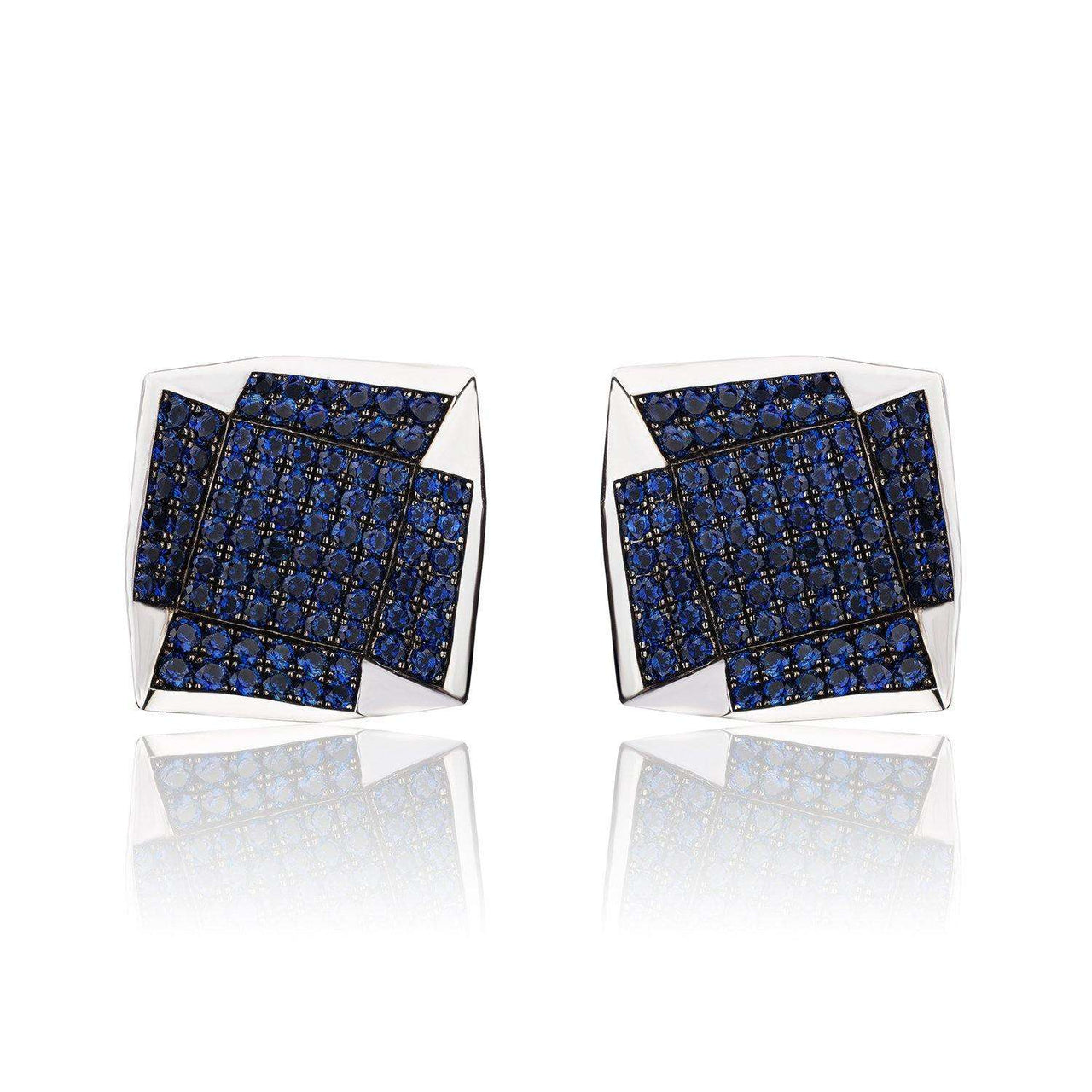The image features two intricate, white fabric cuffs with ornate blue beadwork and subtle silver accents arranged in a grid pattern. These cuffs are reflected symmetrically, creating the illusion of being placed on a reflective surface, despite not sitting on any physical surface. The beadwork includes a detailed blue box design that appears to spread open in the middle. The background is a stark white void, enhancing the contrast and visibility of the cuff designs. The image seems to have a stylized graphic presentation, suggesting perhaps that the cuffs could be part of a broader repeat pattern that might be used to construct a cubic shape. The main design elements highlight navy and yellow hues, with a possibility of light effects in the corners, and the pattern implies a three-dimensional perspective akin to cube construction templates.